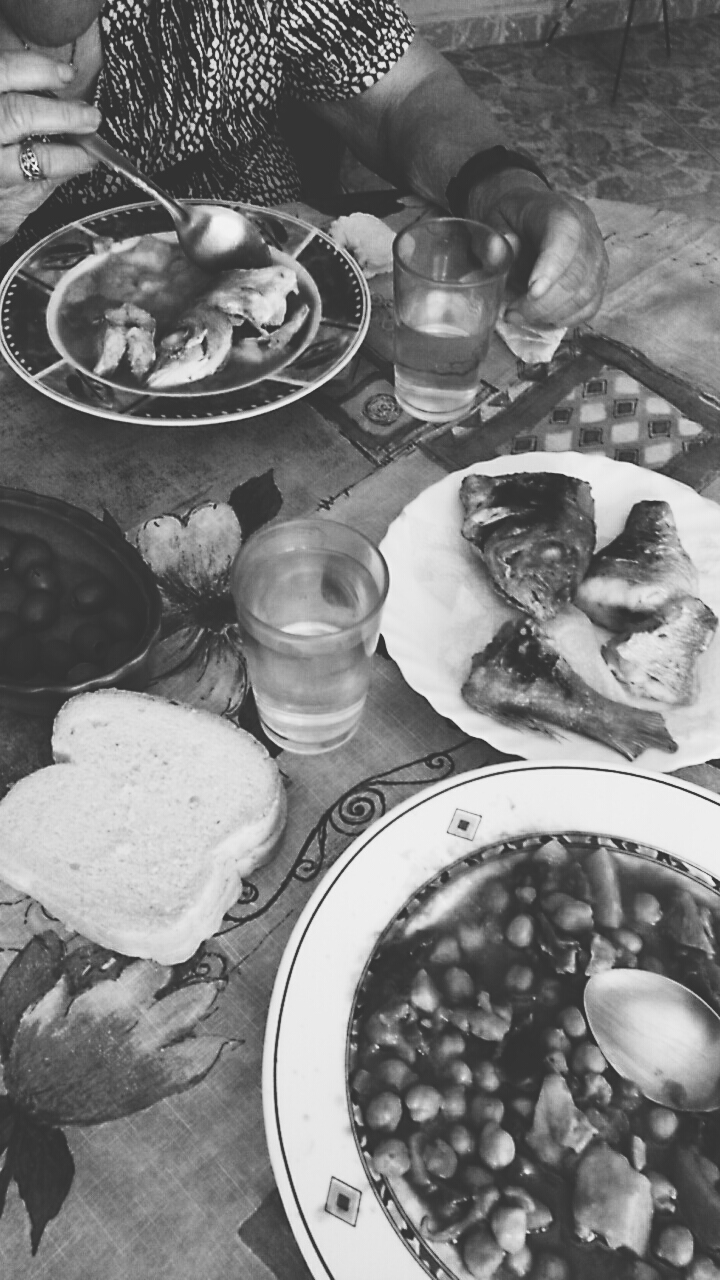The black and white image captures an overhead view of a round table draped with a detailed tablecloth or possibly featuring etchings. Centered in what appears to be an indoor kitchen, the scene is bustling with various plates and bowls of food, indicating a communal meal. On the table, there are clear glasses of water, slices of white bread, chicken wings, pastries, and a bowl that might contain Brussels sprouts or other legumes. One white plate holds an unusual mixture of meats, including what might be fish heads or pig legs, alongside olives and a bowl of soup with vegetables. Occupying the upper left corner, a person dressed in a patterned black and white shirt, identifiable by their ring and watch on their left hand, is actively eating with a spoon. While the overall setting feels vibrant and inviting, the monochromatic palette adds a timeless touch to this richly detailed culinary spread.